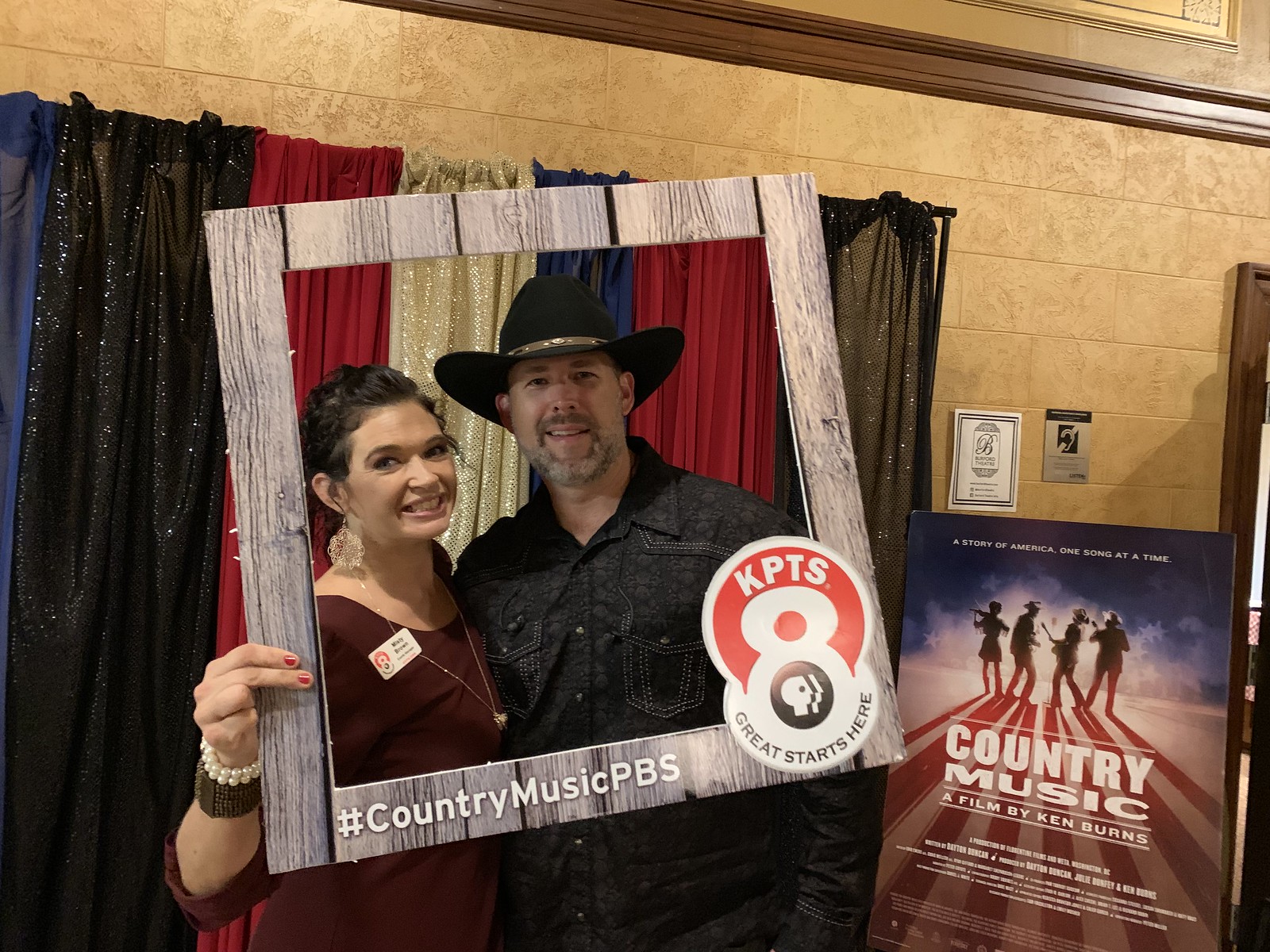In the image, there is a man and a woman standing inside a room against a backdrop of vertically hanging curtains in alternating colors: black, red, gold, blue, red, and black. The wall behind the curtains is stone-textured, made up of horizontal rectangles. The woman, positioned on the left, is holding a large picture frame that makes it look like their upper bodies are inside the frame. The bottom of this frame reads "KPTS 8" and "Great starts here," with a hashtag "#CountryMusicPBS" on the left.

The woman is a white female with brown hair pulled back. She is wearing a short-sleeved dark red or maroon shirt, a silver necklace, large round earrings, and a name tag. She is smiling at the camera. The man, standing to her right, is a white male with thin facial hair that is partly gray and brown. He is wearing a black cowboy hat and a dark denim, long-sleeve button-down shirt with sparkly designs. 

To their right, there is a sign featuring the silhouette of four musicians, with text that reads: "Country Music" in bold white letters, "A Story of America One Song at a Time," and "A film by Ken Burns."